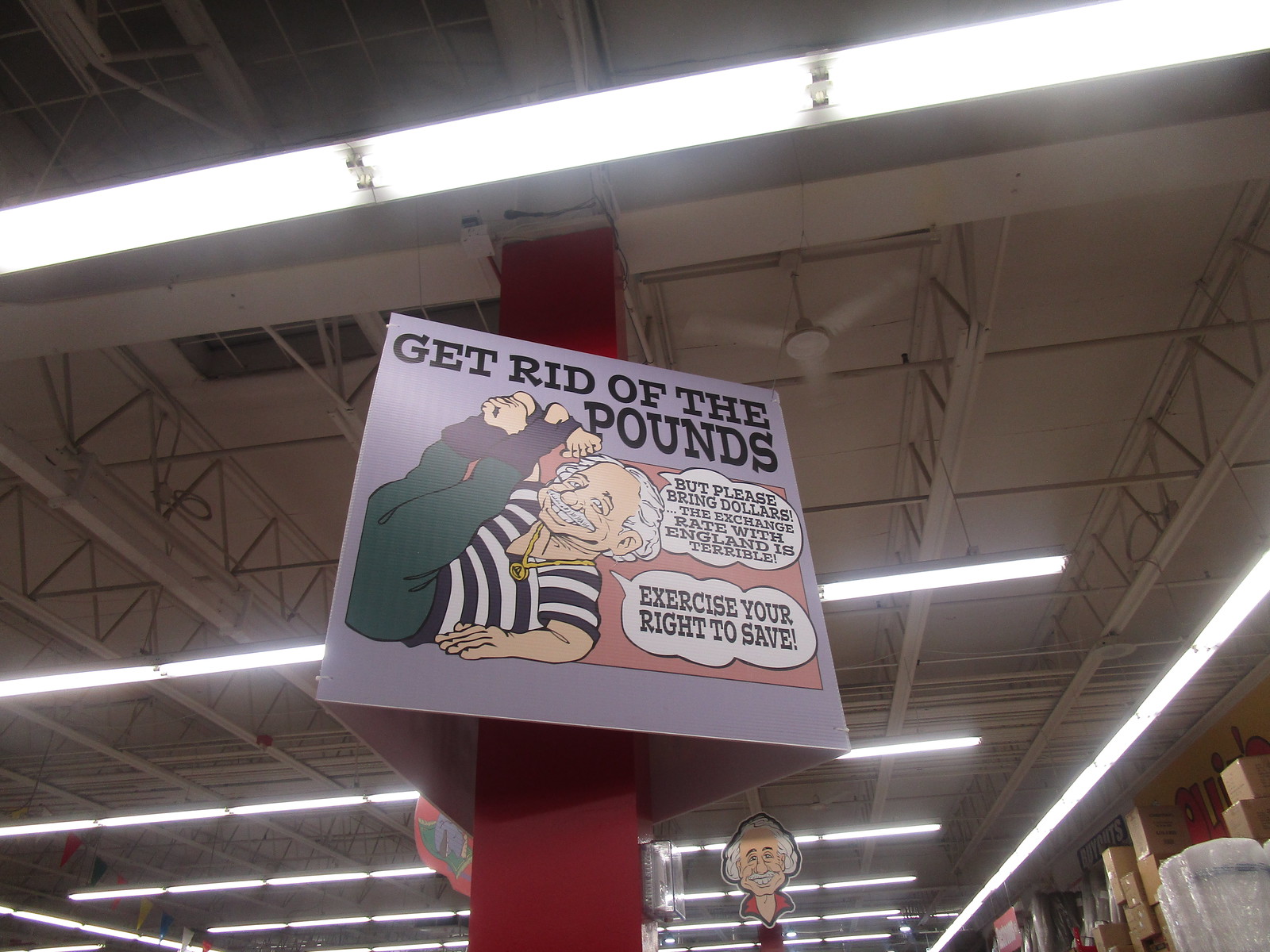This photograph, taken from below, captures the ceiling of a large industrial building or warehouse, featuring long rows of fluorescent lights stretching into the background alongside structural materials like fans. Dominating the foreground is a prominent red rectangular post, which holds a three-sided purple sign. The visible side of the sign depicts a cartoon-like figure reminiscent of Albert Einstein, identifiable by his balding head with white hair, white mustache, and gold chain. The man is depicted lying on a pink carpet with his legs raised and grabbing his feet, smiling as he appears to exercise. The sign reads, "Get rid of the pounds, but please bring dollars. The exchange rate with England is terrible," and "Exercise your right to save." Additional speech bubbles, although unreadable, emanate from the character. The man's face is also repeated at the bottom right of the image. In the background, beyond the post, are tall shelves stocked with various boxes, some orange and others plain cardboard, hinting at the warehouse function of the space.